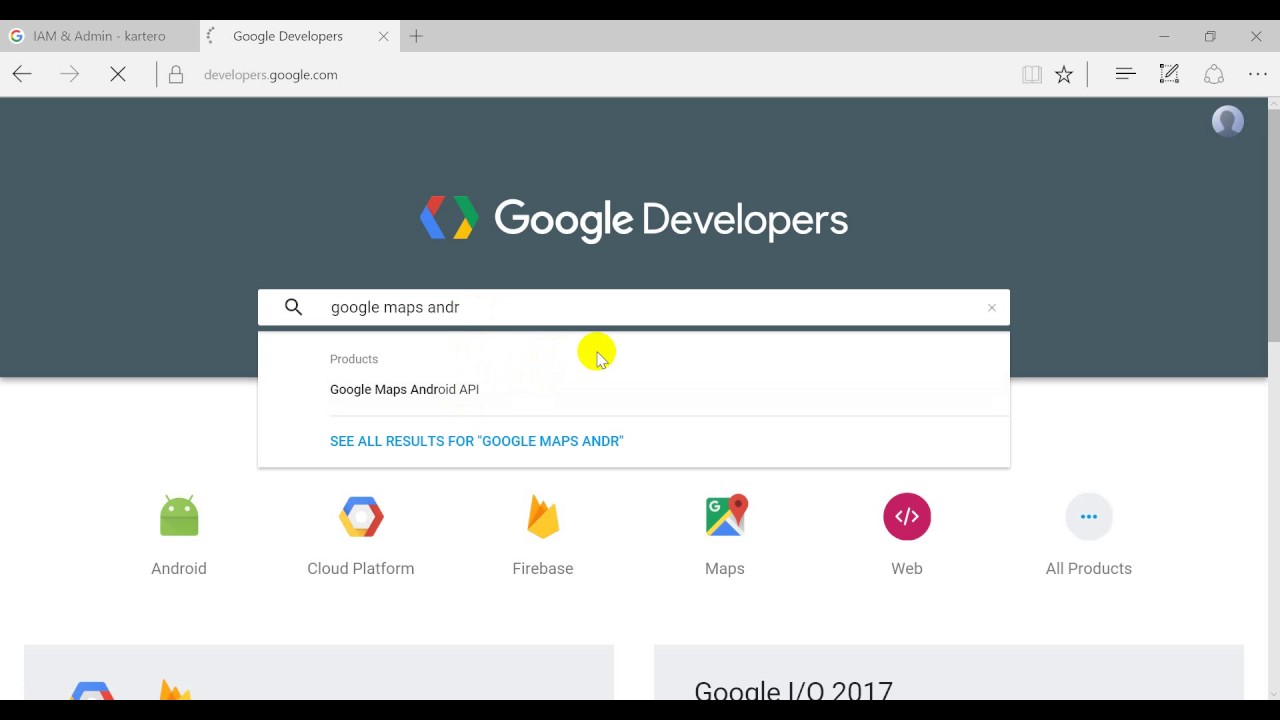This image is a screenshot from a computer, presented as a horizontal rectangle. At the center, against a gray background, the text "Google Developers" is prominently displayed, accompanied by a colorful diamond-like symbol to the left. Below this, there is a white search box featuring a magnifying glass icon on the left and pre-filled with the text "Google Maps ANDR," indicating a search for terms related to Google Maps and Android.

Underneath the search box, the text suggests that the query is looking for "Google Maps ANDROID API" with a prompt to "See all results for Google Maps ANDROID."

Further down, within a white section, several symbols and labels are presented in a row:
- A small green alien icon labeled "Android"
- A colorful hexagon labeled "Cloud Platform"
- A fire symbol labeled "Firebase"
- A map icon labeled "Maps"
- A pink circle with arrows labeled "Web"
- A gray circle with three dots labeled "All Products"

This page is evidently a resource hub for Google Developers, specifically aimed at those looking to develop applications or services for Google's Android platform.